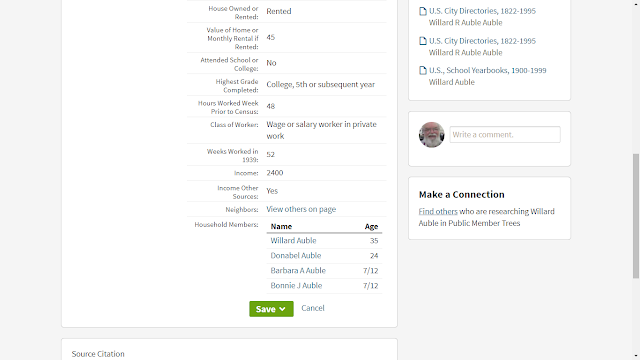This image depicts a well-organized real estate-related website interface, featuring comprehensive information centered on household details. The main content is displayed within white boxes contrasted against a gray background. At the top, the interface lists several categories of information. It begins with the dwelling details, "House Owned or Rented: Rented," followed by financial information, "Value of Home or Monthly Rental if Rented: $45."

Next, it covers education status, addressing "Attended School or College: No" and "Highest Grade Completed: College, Fifth or Subsequent Year." Employment details are highlighted with "Hours Worked Prior to Census: 48," "Class of Worker: Wage or Salary Worker in Private Work," "Weeks Worked: 52," and "Income: $2400." Additional income is noted with "Other Income: Yes." Below these, there's an option to view more information with "View Others on Page."

The interface also lists household members, noting that there are three. Below this information, a prominent green "Save" button is available for user interaction.

On the right side of the page, there are sections for historical records: 
- "U.S. City Directories, 1822-1995" listing one of the household members.
- Another similar entry for "U.S. City Directories, 1822."
- A distinct entry for "U.S. School Yearbook, 1900-1999," listing the main person.

Additionally, there's a box displaying an image of the main individual, described as a white man with a white beard and mustache. Beneath this, users are prompted to "Write a Comment" and explore further interactions with options under "Make a Connection," to find others researching "Willard, Olival, and Public Member Trees."